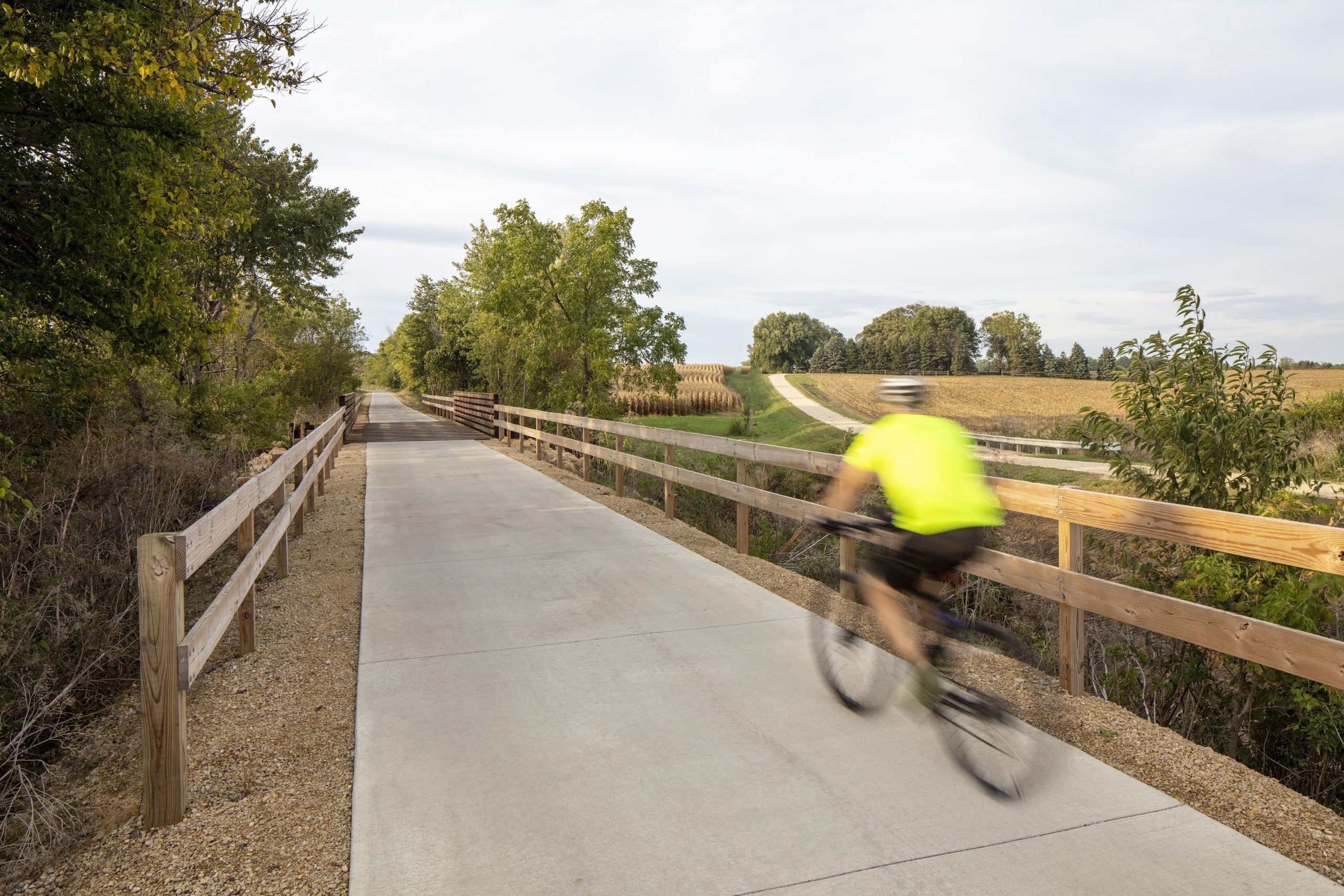The outdoor photograph, captured in landscape layout, depicts a man riding a bike on a wide concrete path that extends diagonally from the bottom right to the top left of the image. The cyclist, who is a blur due to motion, is wearing black shorts, a neon lime green shirt—resembling a highlighter for visibility—and a helmet. His bike is black. 

On either side of the path are wooden fences, consisting of vertical posts with two long horizontal planks, made from treated light brown wood and bordered by mulch. The left side of the image features dense, leafy green trees, while the right side shows a mixture of greenery, grass, and a brown field extending into the distance. In the far background is another path or road with a silver guardrail that suggests it might connect with the main path. The sky overhead is a blend of grayish-blue with some white clouds, adding a serene backdrop to the scene.